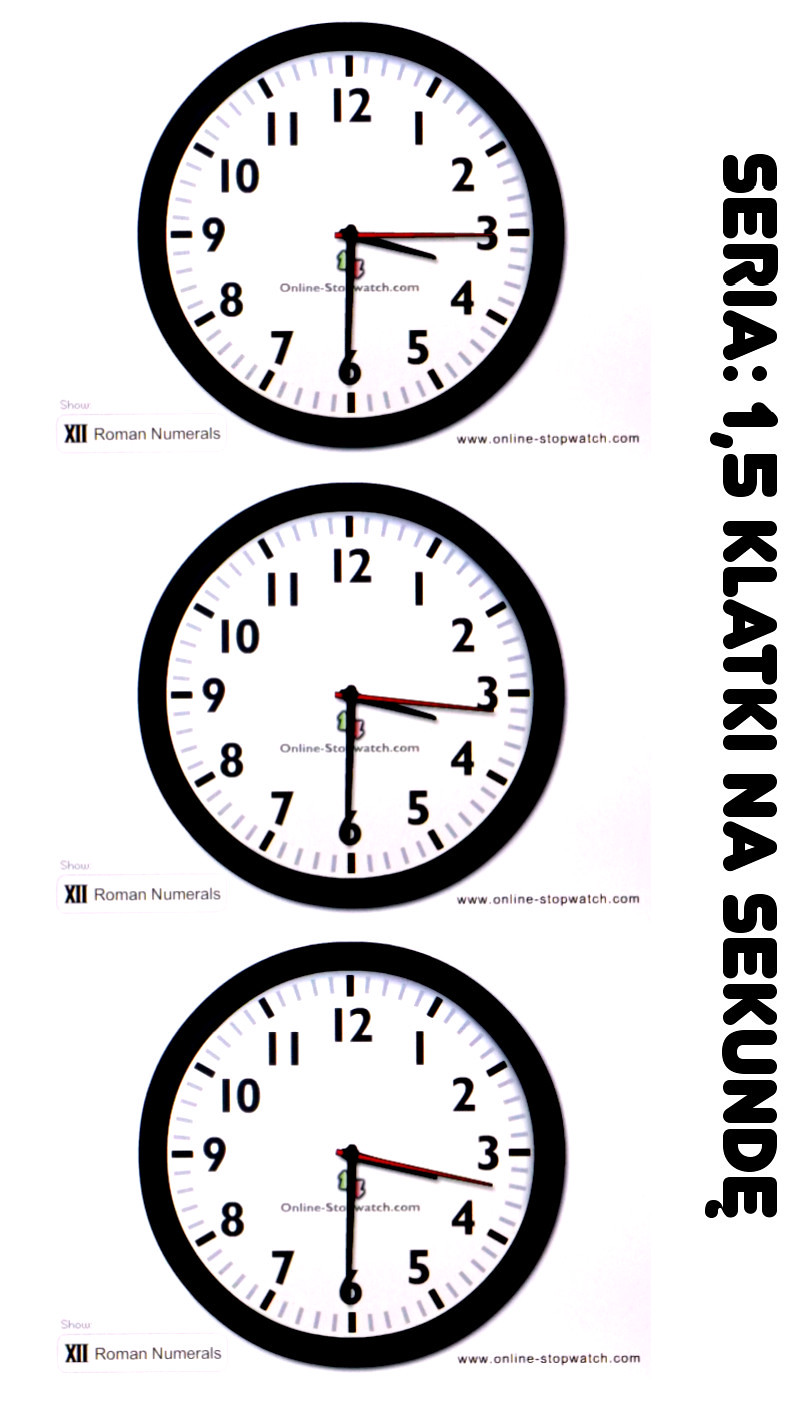The image is a mostly black and white photograph featuring three circular wall clocks arranged vertically in a column. Each clock face is encased in a black round outline with black numbers indicating the hours and minutes. The clocks uniformly display the time as 3:30, but their red second hands differ slightly. The top clock’s second hand points to the third second, the middle clock’s to the sixteenth second, and the bottom clock’s to the seventeenth second. On the left side of the image, there is black text that reads "SERIA: 1, 5, KLATKINA, SECUNDE". Below each clock face, the Roman numeral "XII" is displayed, and the URL "www.online-stopwatch.com" is visible near each clock face.